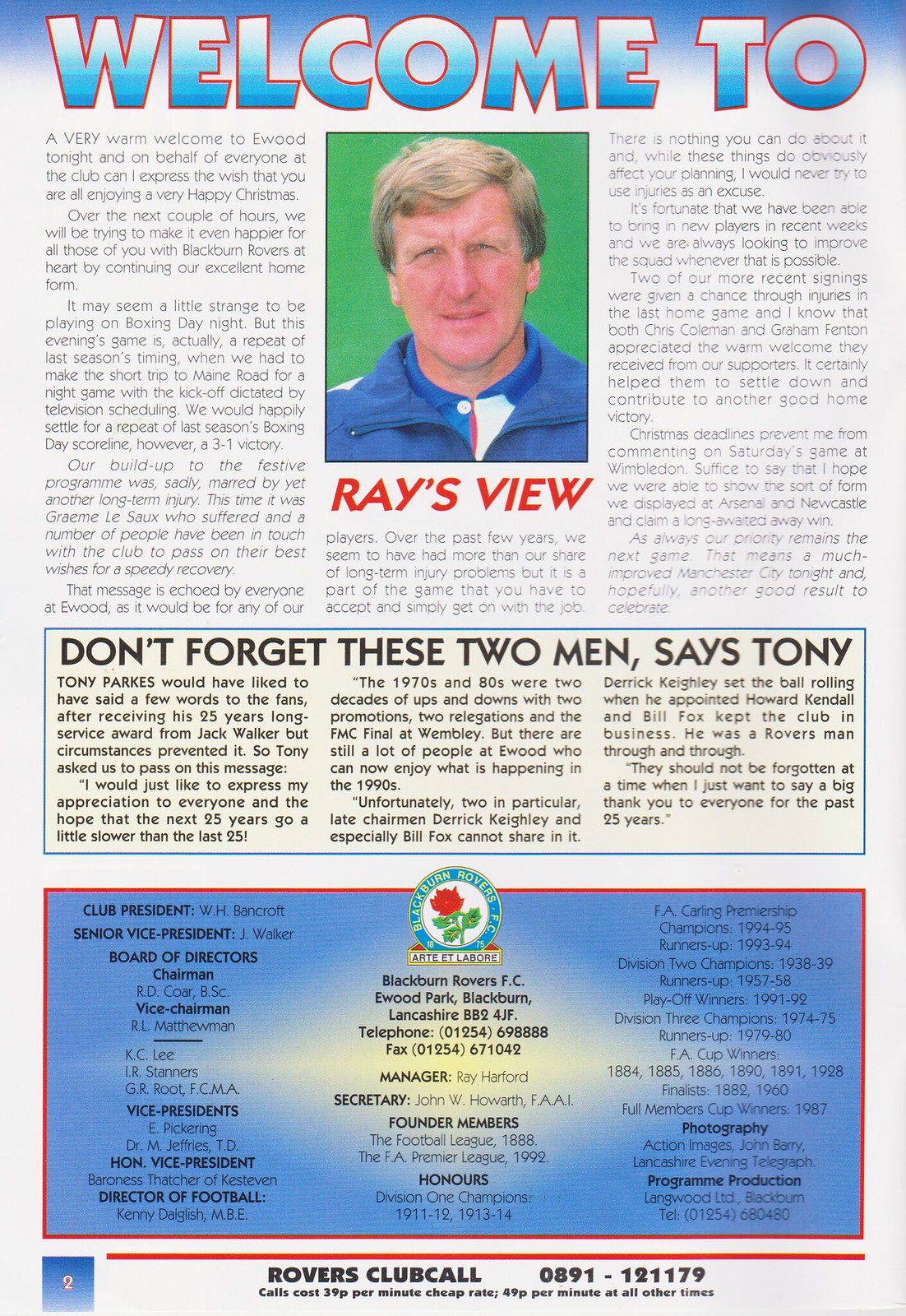The image depicts a page that appears to be from a magazine or newspaper, specifically focusing on a European soccer club, Blackburn Rovers. The layout features a white background with a mix of text boxes and images. At the top of the page, there is a heading that reads "Welcome to Ray's View," accompanied by a photo of a man identified as Ray, who is presumably the author of the article. Ray, a blonde, white man in a blue shirt, is set against a green background, with his section title "Ray's View" highlighted in red letters.

Centrally located on the page is a blue-bordered text box with bold, black font that states, “Don’t forget these two men,” followed by a message from someone named Tony. This section emphasizes important individuals related to the soccer team. Surrounding this highlighted box are two columns of text detailing updates and information about the Blackburn Rovers, including recent activities and relevant news about the club.

The lower section of the page features another blue text box bordered in red, providing comprehensive information about the club's organizational structure. This includes the names of the club president, WH Bancroft, senior vice president, Jay Walker, other board members, and additional roles such as managers and secretaries. It also lists records of championship wins and credits for photography and program production. Additionally, the bottom part contains several contact numbers and advertisements, concluding with "Rovers Club Call 0891-121179." The overall design contains a mix of blue, red, and black text elements, creating a visually appealing layout for the readers.